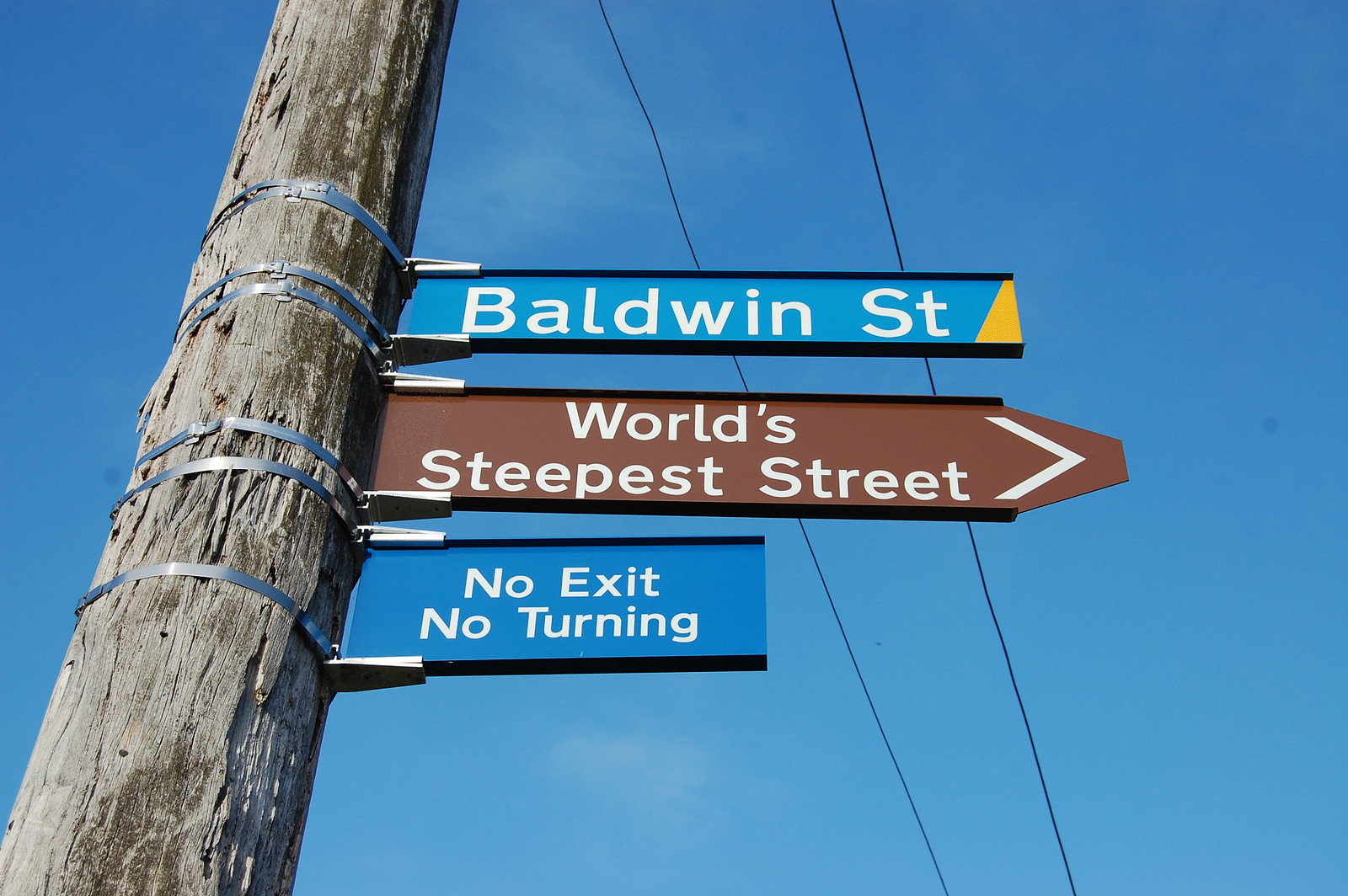In a photograph taken on a bright, sunny day featuring a clear, azure sky devoid of any clouds, a grayish-brown wooden pole stands prominently on the left side of the image, slightly angled to the right. Affixed to the pole with chrome-colored metal bands, three distinct street signs extend to the right. The top sign is a narrow blue rectangle adorned with a gold triangle on its far right edge, displaying the words "Baldwin Street" in white type. Below it, a brown rectangular sign with a blunt point on the right edge reads "World's Steepest Street" in white type. The bottom sign, rectangular and shorter than the others, is blue and bears the message "No Exit No Turning" in white type.